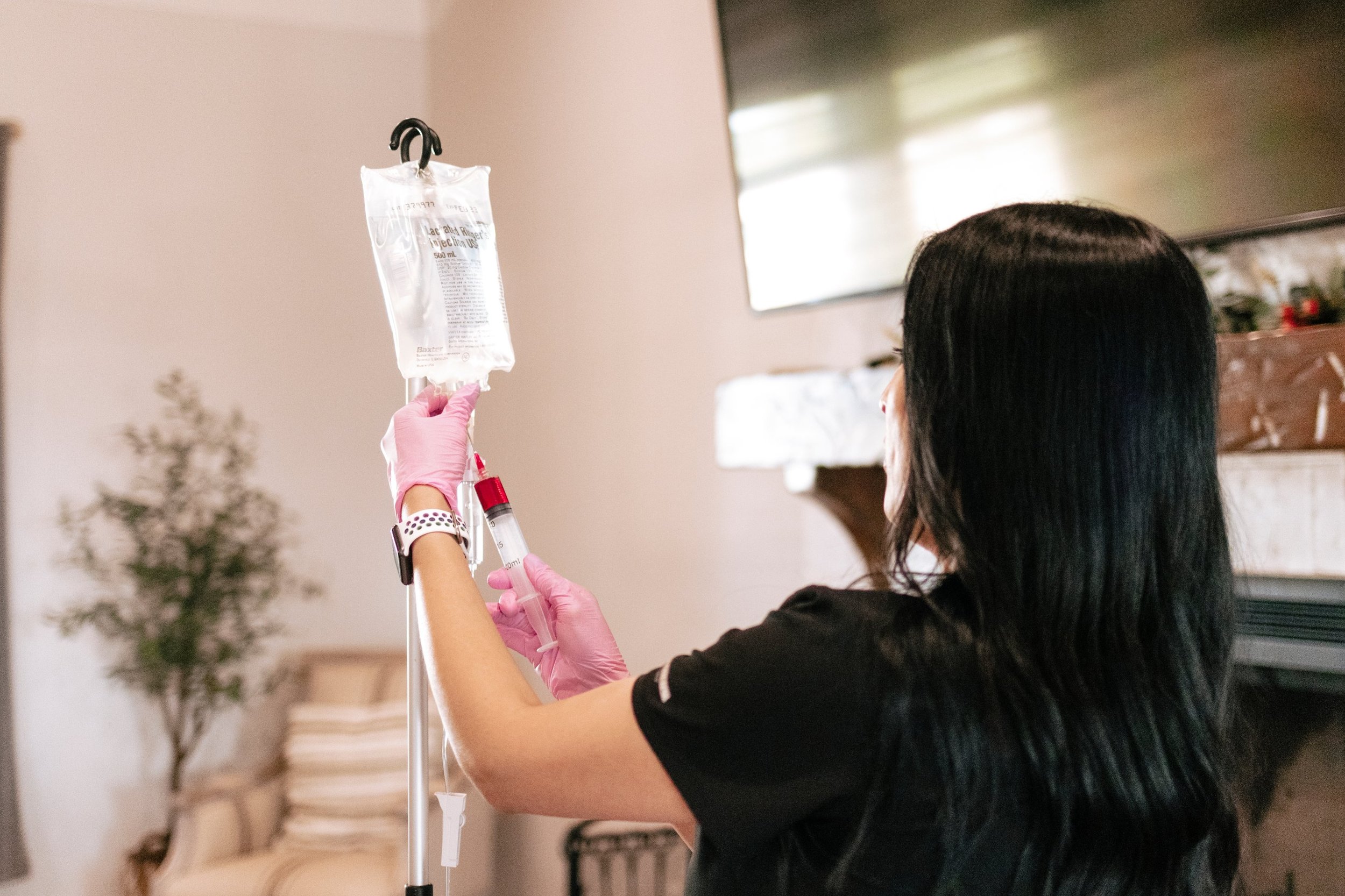In the image, a woman with long, dark black hair, wearing a black t-shirt and pink rubber gloves, attends to an IV bag. She is positioned on the right side of the picture, facing away from the camera. She holds a syringe filled with red liquid in her right hand, and dons a white watch on her left wrist. The room appears somewhat domestic rather than clinical, with a beige and light brown chair, a small potted tree, and a white wall on the left side. Adding a touch of ambiguity, a large flat-screen TV is mounted on a wooden mantel above a fireplace on the right. The bright lighting enhances the clear details in the image, suggesting she might be a nurse performing a medical procedure, evident from her focused handling of the IV setup. Despite the medical activity, the warm and homely background contrasts with the clinical task she is performing.